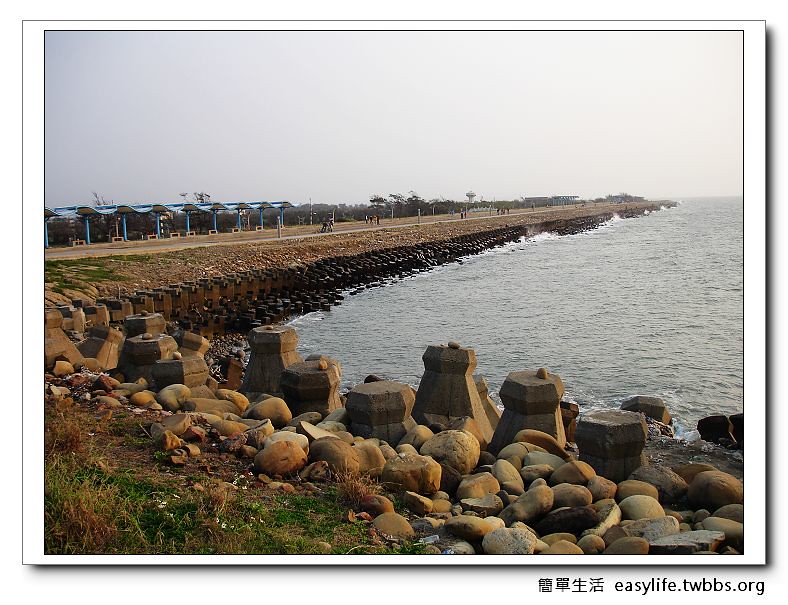A large body of water occupies the right half of the image, presenting a slightly wavy, grayish surface with splashes against a protective barrier made up of barrel-like objects. These barriers separate the water from the land, where rocks and grass are visible, leading to a sidewalk where several people stroll. On the left towards the middle, there is a rest area shaded by a light blue canopy supported by several blue posts, likely providing a place to sit. Trees form a backdrop in this area, extending to the back. The foreground features an assortment of stones of various shapes and sizes, adding texture to the scene. A long, brown rocky road stretches out into the waterway from the back left, reinforcing the landscape's connection with its aquatic surroundings. The photo is attributed to the Easy Life Twibs organization, as noted at the bottom right of the image.